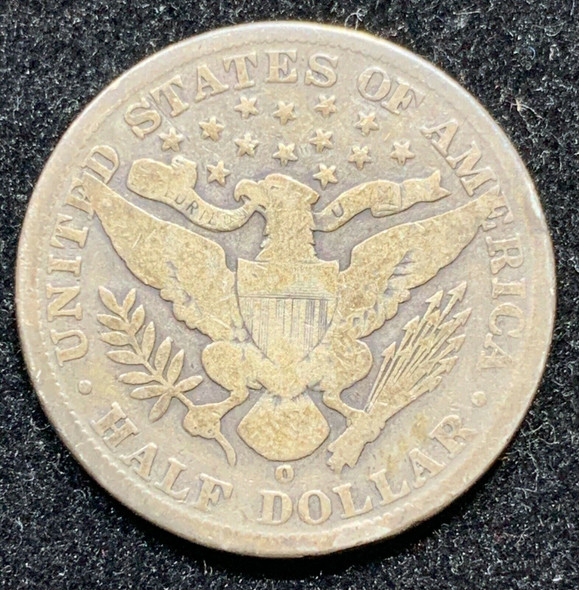This image features a close-up photograph of a United States of America half dollar coin set against a gray, granite-like background. The coin itself has a bayish or light copperish tone, with raised decorative lettering around its outer edge. At the top of the coin, the words "United States of America" are inscribed, while "Half Dollar" is written at the bottom.

Central to the coin's design is a stylized eagle with extended wings. The eagle is adorned with a shield on its chest, which features vertical bars and a bayish or copperish hue at the top. The eagle clutches an olive branch with its left talon and a bundle of 13 arrows with its right, symbolizing peace and strength. In its beak, the eagle holds a banner reading "E Pluribus Unum." Surrounding the eagle's head are 13 stars, representing the original colonies. Below the tail of the eagle, a small, indistinct mark resembling a zero or an "O" is visible. The coin's surface exhibits a worn, spotty appearance, revealing hints of both gold and silver hues through areas of rubbing and fading.